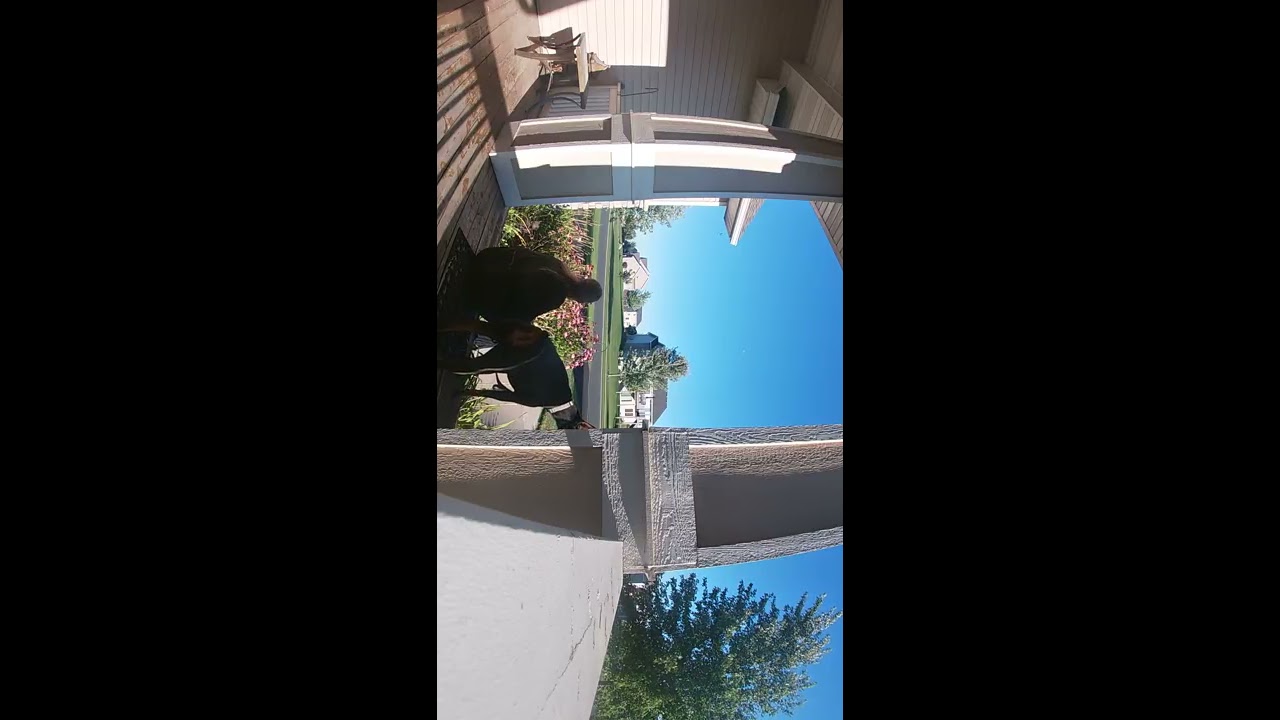This sideways-oriented photograph appears to be taken from a deck or porch attached to a wooden house with light brown and beige hues. The image is slightly warped, hinting it might be from a doorbell camera, making the horizon and scene somewhat disoriented. Despite the orientation, we can discern the deck is supported by two wooden columns reaching up to the roof, with the deck's surface featuring a mat.

Center stage, a large dog, likely a Doberman wearing a white collar, stands partly obscured behind one of the columns. Next to the dog, on the left, sits a shadowed individual, whose features are difficult to make out. To the left side of the deck, there is a table adding to the porch's furnishings.

The background reveals a picturesque view with a clear blue sky and various natural elements. Trees, bushes, and a road extend outward from the decking area. Across the street, there are several similarly styled two-story houses, nestled among more trees. One prominent feature is a large pine tree on the right. Further into the distance, you can observe a large white house, a barn-like structure with a tree in between, and a quaint farm-like scene, completing this serene outdoor setting.